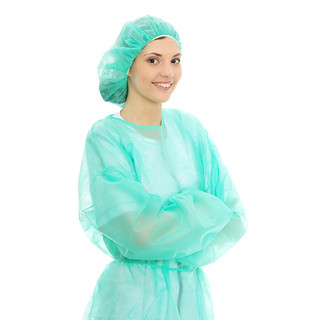A woman stands facing slightly to her right, her head turned towards the camera, showcasing her smiling face. She is wearing a white T-shirt and white pants, covered by a teal green, semi-transparent netted gown which features an elasticized waist that pinches in slightly, causing the material to flare out around her. Her brown hair is pulled back and tucked under a matching teal green hairnet, although a small portion of her hairline is visible at the front. The mesh material, loosely draped over her form, creates a series of bulges and wrinkles. Her arms are crossed over her chest, projecting confidence. This appears to be a staged photo, likely for a modeling or medical-related context, with a seamless, photoshopped background that emphasizes a clean and clinical aesthetic. Despite the protective attire, she wears light makeup and has a neat, polished appearance.